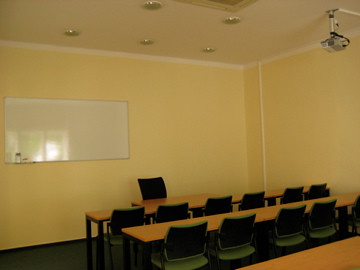This detailed caption describes a color photograph of a room that resembles a classroom or a presentation room. The room has pale yellow walls and a white ceiling adorned with five recessed light fixtures. Centered between the floor and the ceiling on the back wall, to the left of the image, there is a whiteboard. Below this whiteboard, a desk with a larger black chair faces the front, suggesting a teacher or presenter’s area. Three long, rectangular tables with brown wooden tops are neatly arranged in rows to the right. The middle table has four green chairs with black backs, while the table closest to the wall has six similar chairs and a laptop sitting on top. Additionally, there is a gray overhead projector suspended from the ceiling with black wires protruding from it, indicating the room’s capability for audiovisual presentations. The floor appears to be covered with black, flat institutional tile or heavy carpeting.